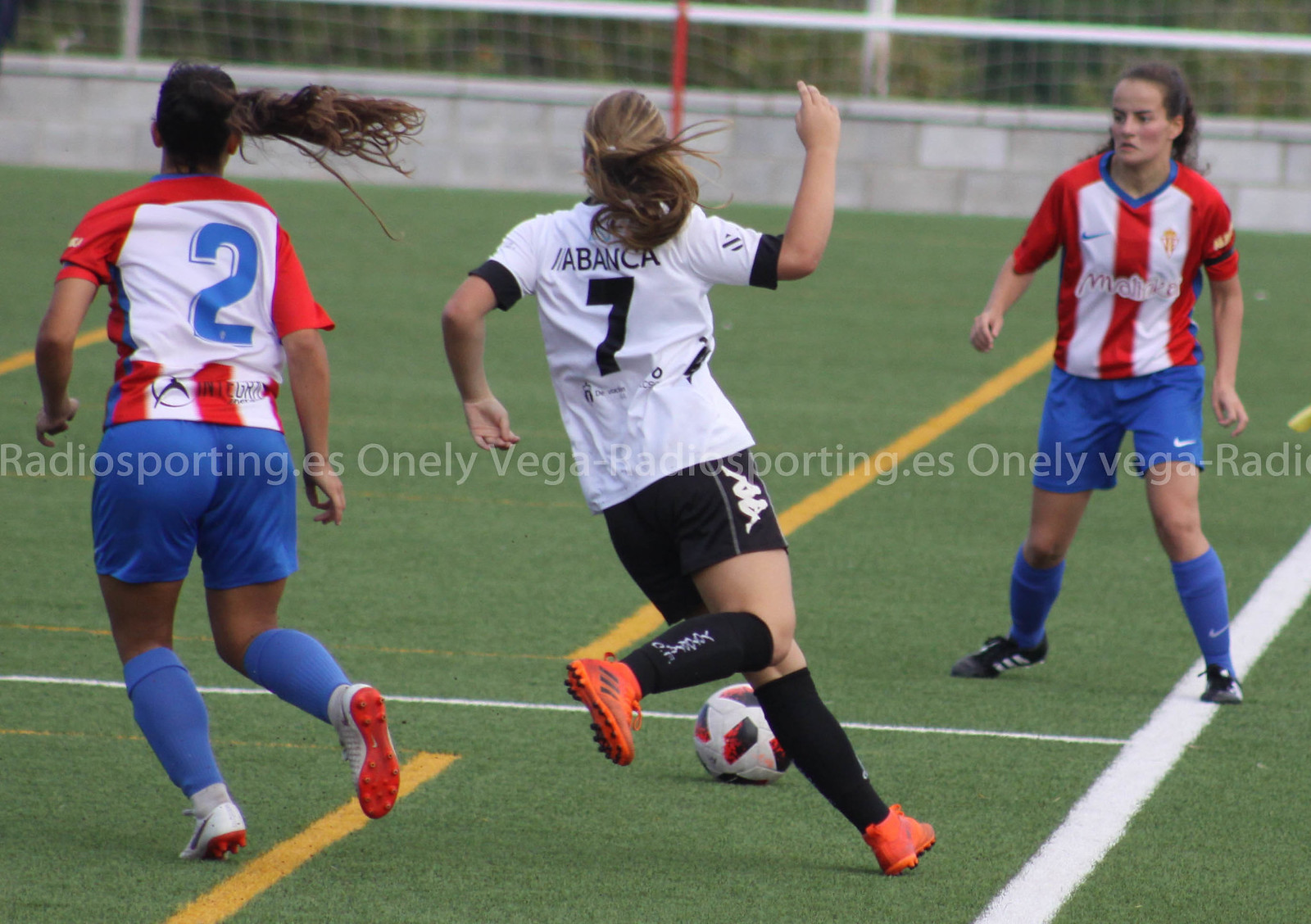In this vibrant outdoor image capturing a dynamic moment of a women's soccer game on an artificial turf field, we see three determined competitors. The player on the left, with long dark hair tied in a ponytail, is in mid-run, her back towards us. The middle player, with slightly lighter hair also in a ponytail, is poised to strike the ball in front of her—a white ball with black and red patches. She is dressed in black shorts, black socks, neon orange cleats, and a white top with a black number. To the upper right, a third player in a red, white, and blue uniform is intensely focused on the action. This player, showcasing her front side, is number two; her blue socks and blue shorts complement her red, white, and blue top. The field's green grass is lined with white and yellow markings, and in the background, a wall and a fence border the field, with trees visible beyond. Overlaid faintly across the middle of the image are the words "radiosporting.es, onelyvegaradiosporting," repeating in a subtle pattern.